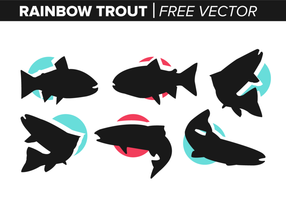The image showcases a collection of six black silhouette vector images of rainbow trout, labeled "Rainbow Trout Free Vector" at the top with a black banner and white, all-caps text. The trout silhouettes are overlaid on colored circles; two turquoise and one red on the top row, and two turquoise and one red on the bottom row. The top row features three trout, while the bottom row includes another three. The fish appear similar in size and shape, with matching fins and tails, organized neatly in rows and columns, and each silhouette has a colorful circle backdrop—blue or pink—highlighting the vibrant and dynamic presentation of these free vector graphics.